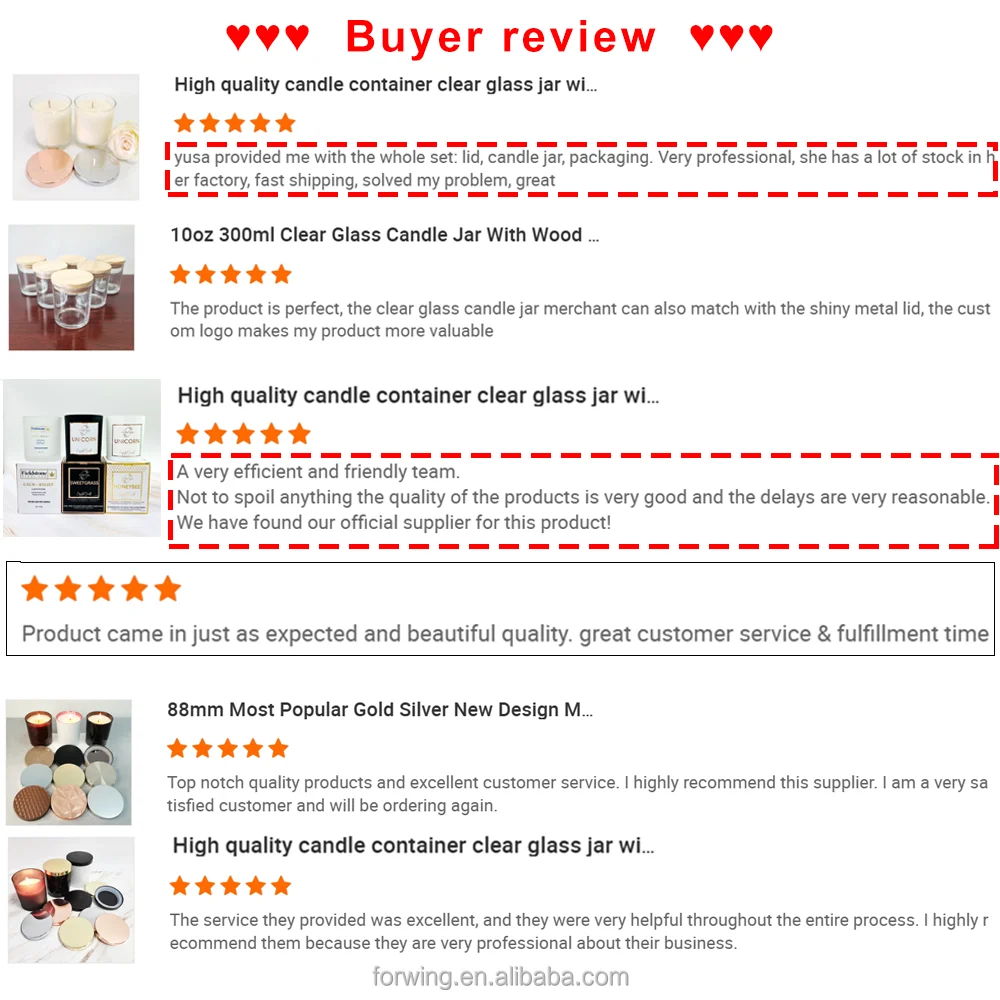This screenshot captures a webpage from 4wing.en.alibaba.com, prominently featuring buyer reviews highlighted in bright red letters with three hearts on each side, centered at the top. The reviews focus on candles and clear glass jar containers. Below are detailed reviews encased in red dashed borders:

1. The first review is for a "High Quality Candle Container, Clear Glass Jar..." with a photo of two white candles. It is rated five stars. The buyer, Yusa, praises the comprehensive set provided, including the lid, candle jar, and packaging. Yusa further commends the supplier's professionalism, ample stock, and swift shipping, all of which resolved their issues.
   
2. The next listing is for a "10 Ounce, 300 Milliliter Clear Glass Candle Jar with Wood," also rated five stars. The review affirms the product's perfection and highlights the added value from the custom logo. The reviewer appreciates the clear glass jar's compatibility with a shiny metal lid, enhancing their product's appeal.

3. Another review for a "High Quality Candle Container, Clear Glass Jar..." rated five stars, applauds the supplier's efficient and friendly team. Emphasizing the excellent product quality and reasonable delivery times, the reviewer states they have found their official supplier for this product.

These reviews collectively affirm the supplier's reliability, product quality, and outstanding service, reinforcing trust for potential buyers.